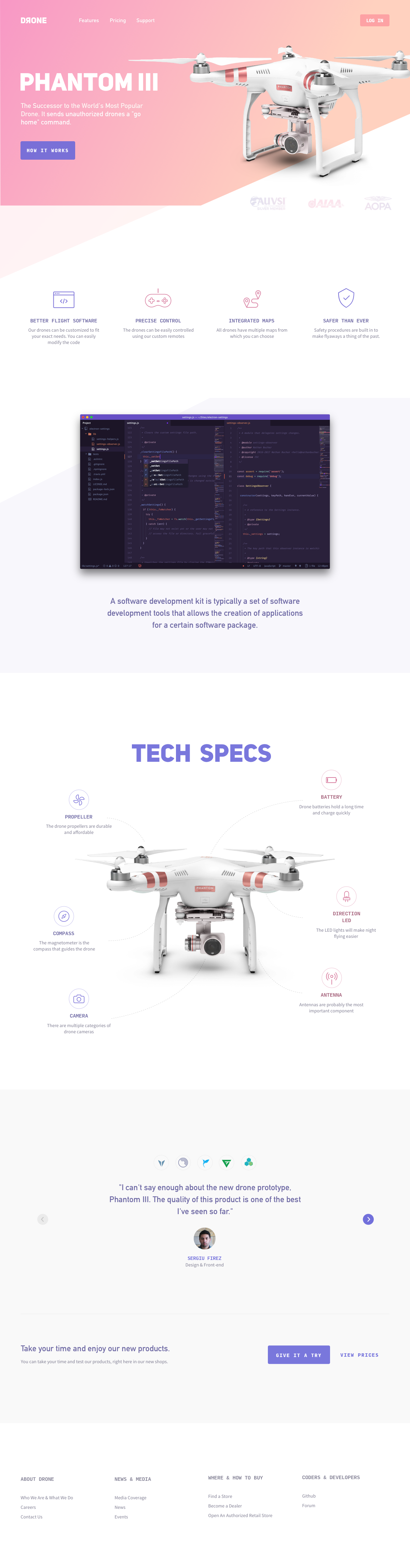This screenshot, taken from an advertisement or poster, features a detailed depiction of the Phantom 3 drone. It outlines an array of technical specifications, including the range of heights the drone can achieve and the advanced programming capabilities built into the device. Notably, the screenshot appears stretched horizontally, making the text somewhat challenging to read.

At the bottom of the image, there is a photograph of an individual with a quotation above it, presumably a review or testimonial about the Phantom 3 drone. Additionally, there is an option to share this review. 

The lower portion of the page includes various navigational titles commonly found on websites, such as "Contact Us." The website’s color scheme is predominantly light, featuring shades of white, slight pink, and purple. The title fonts are rendered in a mix of colors including purple, blue, white, and green.